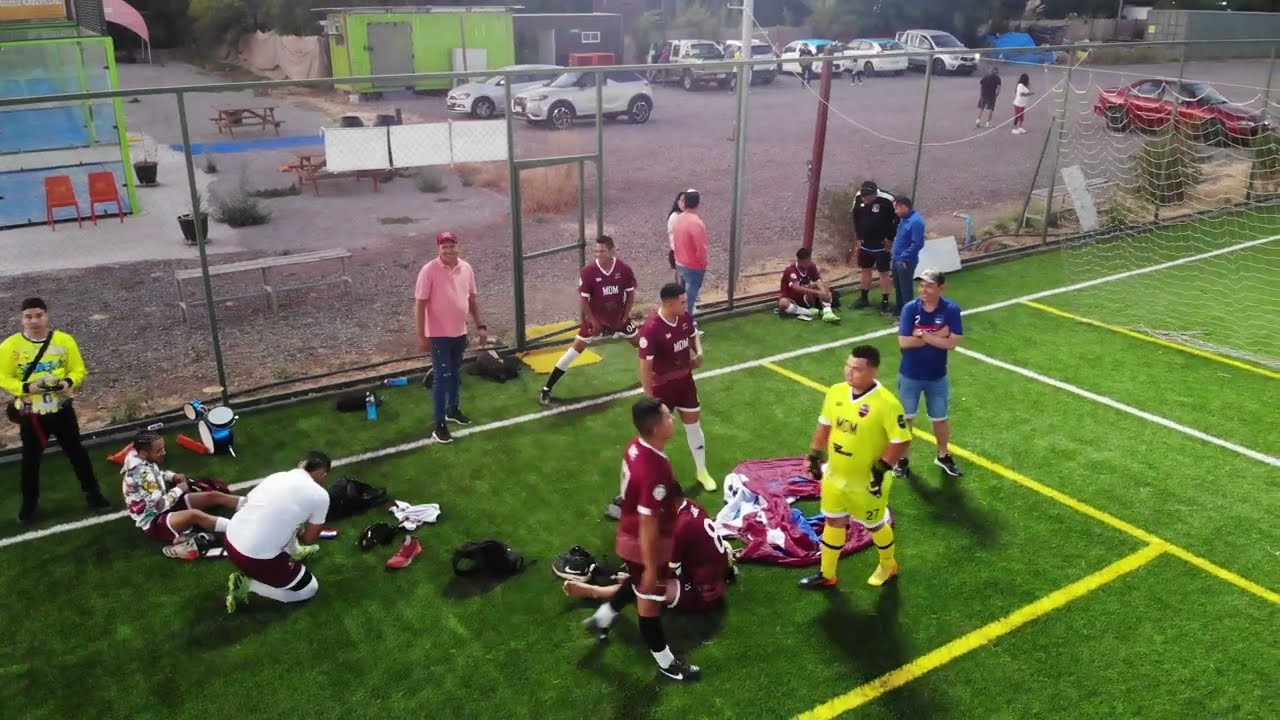The image depicts a vibrant urban soccer field with artificial grass neatly lined with white and yellow markers. In the foreground, the field is surrounded by a tall metal fence, emphasizing its contained environment. Various adults, many dressed in distinct sports uniforms, populate the scene. Notably, one individual stands out in a neon yellow jersey and shorts labeled with the number 27, while the majority of the teammates sport matching burgundy red jerseys and shorts. 

Scattered around the field, several adults are seen in casual clothing, including polo t-shirts, blue shorts, and blue jeans, some preparing for play or sitting down. The lower left corner of the field reveals a more critical moment, where a man in maroon shorts and a white t-shirt tends to an injured player lying on their back, indicating a possible injury.

In the background, beyond the fence, lies a bustling parking lot filled with various trailers and vehicles, providing a stark contrast to the organized activity on the field. The detailed depiction captures the dynamic and multifaceted nature of an urban recreational space in use.